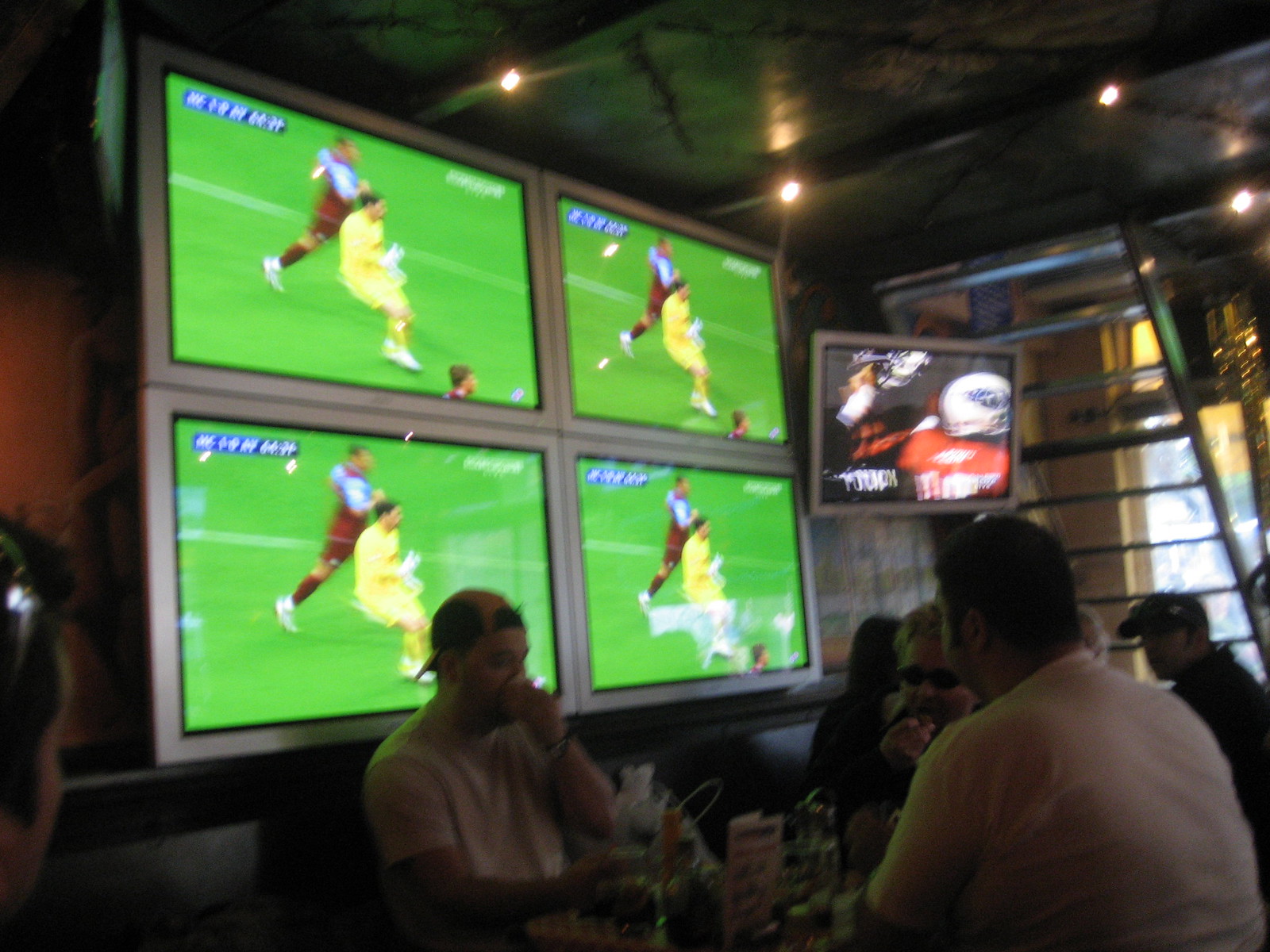In the dimly lit setting of a bustling sports bar restaurant, a lively scene unfolds with patrons eating, drinking, and watching games. At one of the tables, two men are seated across from each other; one, a heavier set man in a white t-shirt with short black hair, is intently focused on the four large TV screens behind his companion. These four screens are bunched together, displaying the same blurry soccer game featuring a player in a yellow jersey and yellow shorts, with another player in a marine uniform with light blue sleeves. Next to these screens, a fifth TV shows an American football game, possibly featuring the Tennessee Titans, albeit unclear.

Nearby, another male patron in a white t-shirt with a hat and a black wristband sits with a man in a black shirt and sunglasses. Their table is cluttered with a menu, drinking glasses, and what appears to be a sauce or soda bottle. In the background, other diners can be seen, including a person rubbing his nose and holding a drink, as well as several more figures relaxing and socializing. A staircase, initially mistaken for a ladder, leads to the second floor, adding to the bar's cozy, multi-level ambiance. The atmosphere is one of camaraderie and sport, with everyone absorbed in the games and each other's company.